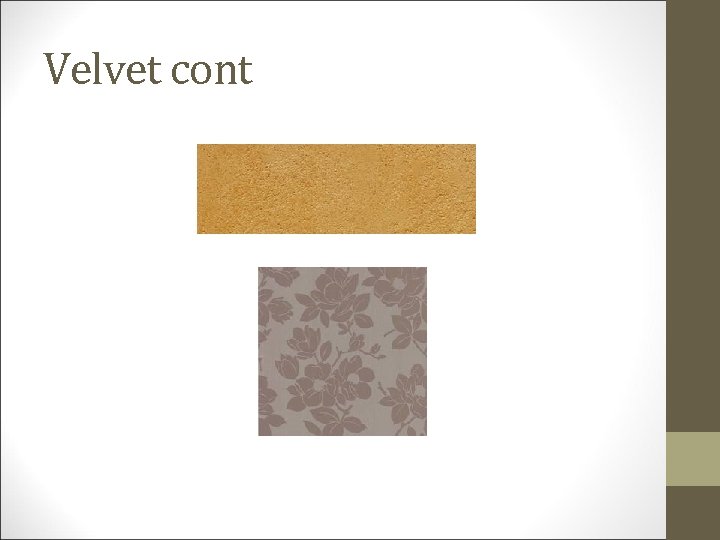The image features a minimalistic design resembling a PowerPoint slide with a white background and some left-side vignetting. Dominating the right side is a vertical dark sage green bar, intersected near the bottom by a lighter sage-colored cube. Inside a large white box are two fabric samples labeled "Velvet cont" (presumably an abbreviation for "continue"). The top fabric sample is a light brown, elongated rectangle with a rough, sandpaper-like texture. Below it, centered, is a smooth, gray square adorned with a dark purple floral pattern on a slightly lighter purple background. The overall composition is framed with subtle text and imagery details, making the fabric textures and color contrasts stand out prominently.